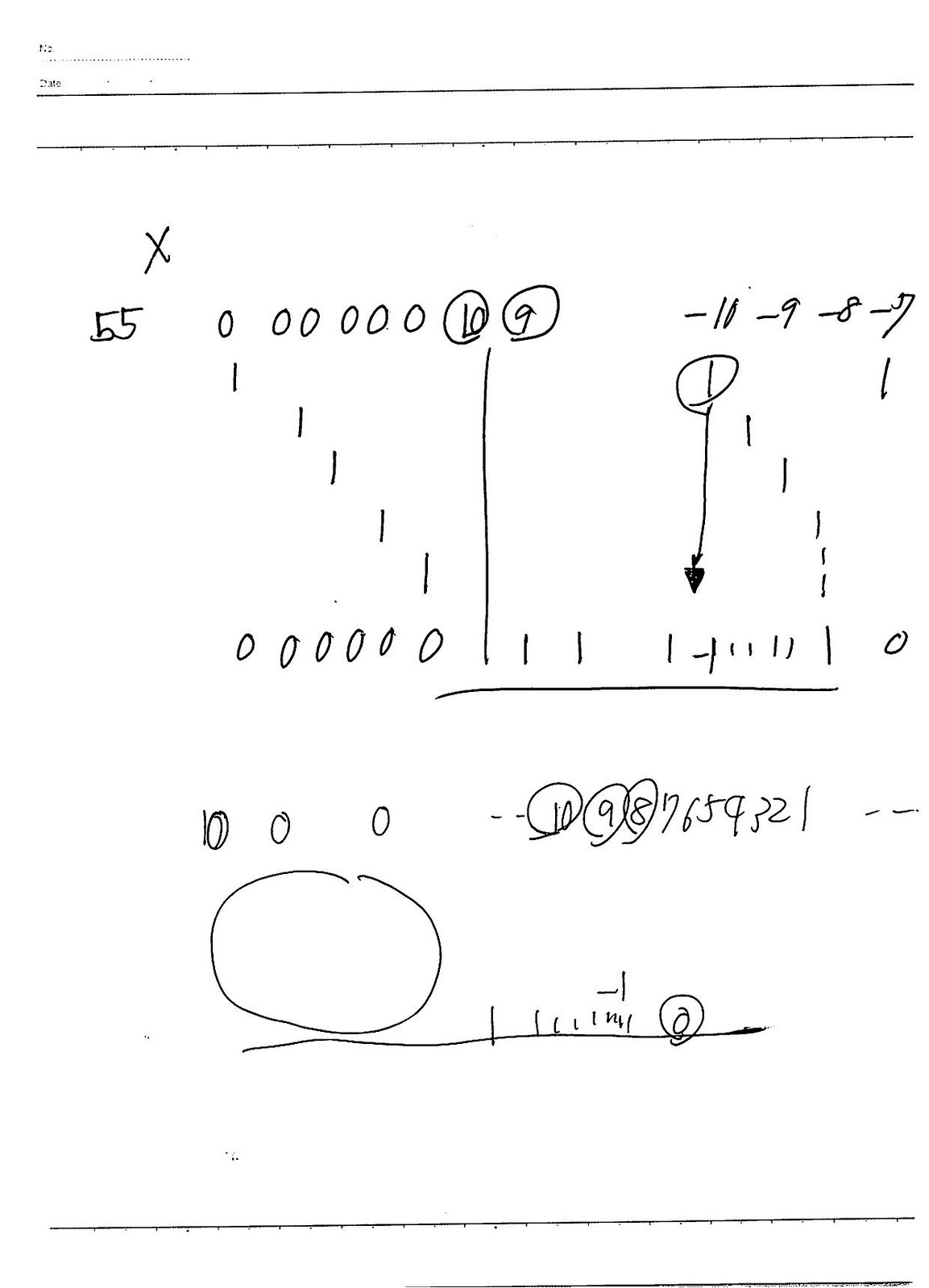A meticulously hand-drawn diagram, rendered in black ink on a pristine white sheet of paper, is captured in this image. At the top of the diagram, two parallel horizontal lines are prominently featured, with the lower line detailed with small etches along its base. Beneath these lines is an array of handwritten annotations. Distinctly visible are symbols such as an "X", the number "55", and a series of zeros. Notably circled are the numbers "10" and "9", situated next to a sequence of decreasing integers: "10, 9, 8, 7".

Flanking this sequence are dashed lines, followed by another series of ones descending from "10" and similarly from "0", which intersect at an angle before forming another array of zeros extending in the opposite direction. Below this intricate setup lies a further sequence of numbers—"10, 9, 8, 7, 6, 5, 9, 3, 2, 1"—with the numbers "10", "9", and "8" again circled for emphasis. The diagram also includes a large "O" or zero positioned over a horizontal line, accompanied by additional scribbles. The composition concludes with two more horizontal lines at the bottom, encapsulating the complexity of the hand-drawn illustration.